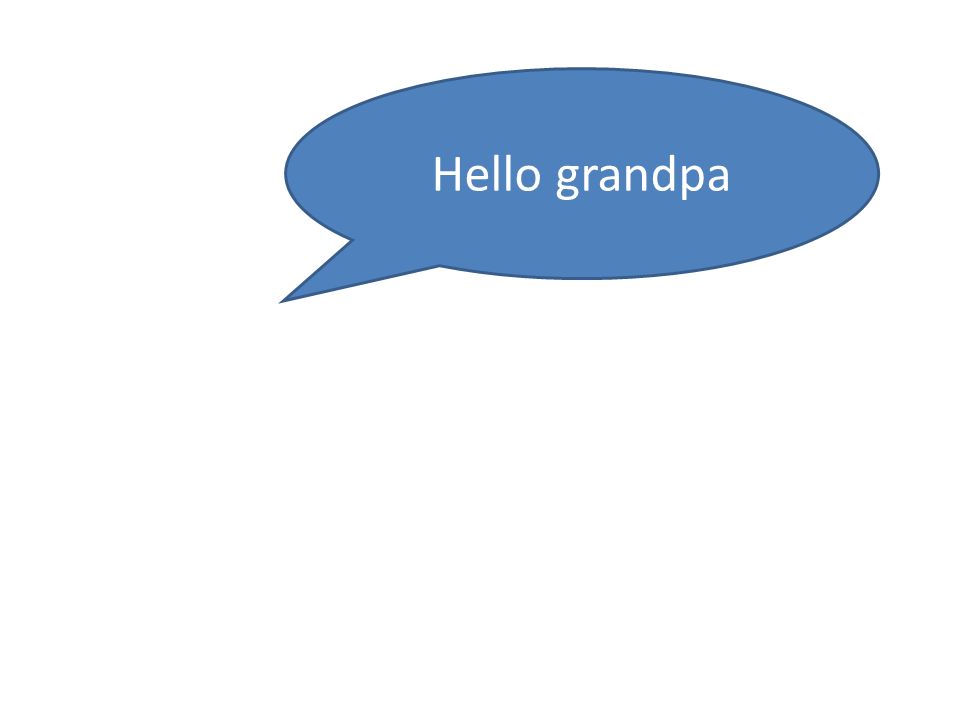The image is a minimalist, comic-style graphic featuring a single speech bubble set against a white background. The speech bubble, which is positioned near the top of the image, is an oval shape with a triangular point extending from its bottom left, suggesting the speaker's direction. The speech bubble is filled with a blue or grayish-blue color, reminiscent of dye blue, and has a darker blue outline. Inside the bubble, in simple white letters, are the words "Hello Grandpa." The text lacks any outlining and shows some JPEG artifacting around it, as well as around the edges of the speech bubble. There are no characters or additional context in the image, leaving the speaker's identity to the viewer's imagination. The overall aesthetic is clean and straightforward, evocative of comic book dialogue bubbles.